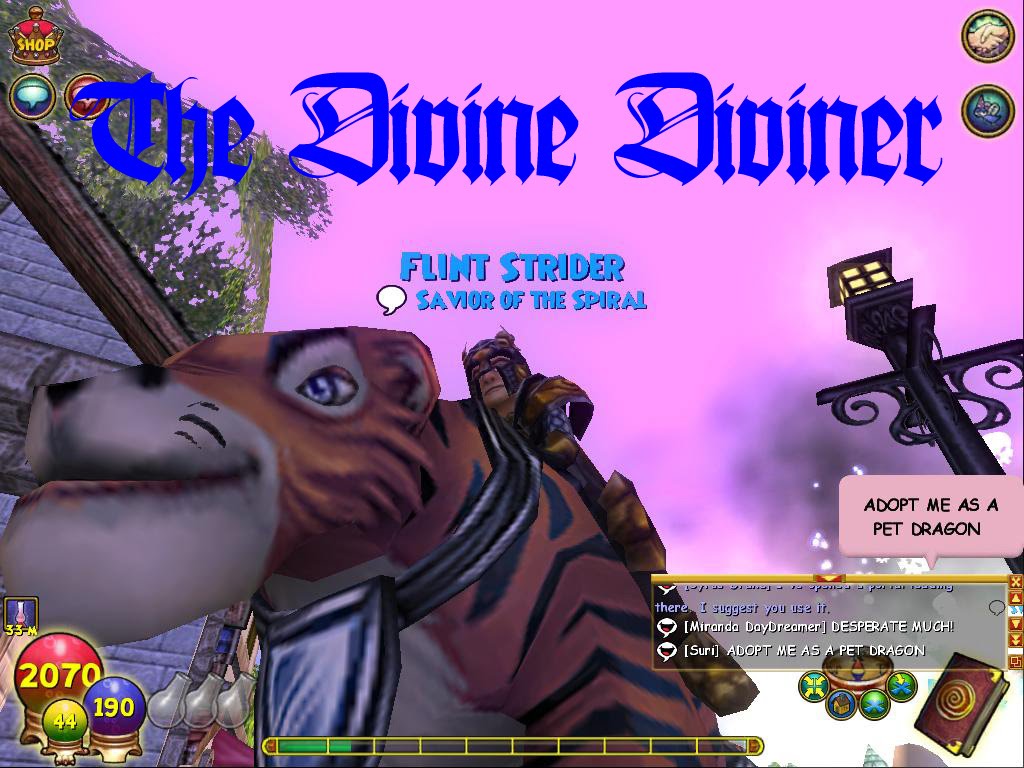The image appears to be a vibrant screenshot from a video game or an online avatar-based game, featuring a striking combination of graphics and text. The background is a bright pink, enhancing the visibility of the ornate text that reads "The Divine Diviner" in blue, with "Flint Strider, Savior of the Spiral" underneath. Dominating the left side of the image is a large graphic of a dragon, on whose back rides a masked man in a costume and boots. Adjacent to this, on the right side, is a black lamppost with a pink text box beneath it stating "Adopt me as a pet dragon." Below, there is a chat box where users Morocco Daydreamer and Surrey are conversing, the latter also asking to be adopted as a pet dragon. The bottom of the image features various graphical elements: a central text bar, a book icon, and a series of spheres on the bottom left displaying numerical values—2070 in red, 190 in blue, and 44 in green.